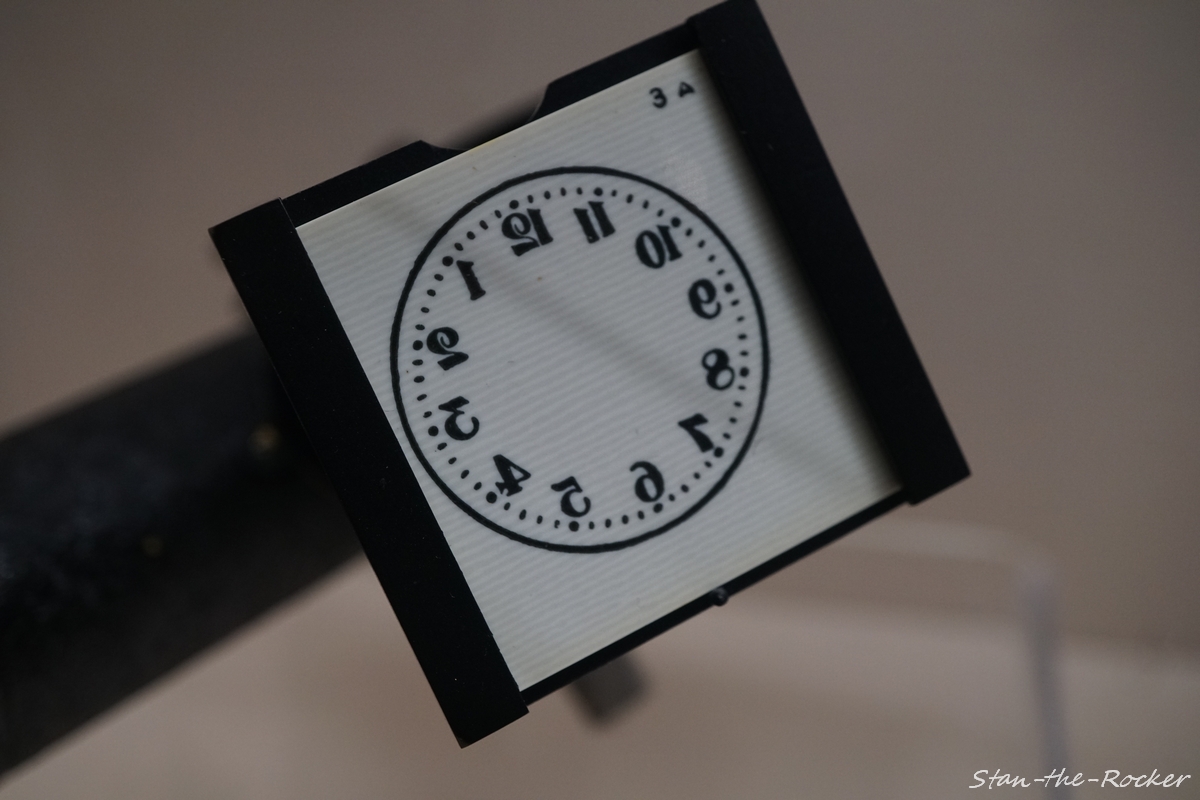The photograph depicts a white sheet of paper displaying an inverted analog clock dial, with the black numbers appearing backward—twelve, eleven, and ten are counterclockwise, with the three on the left and nine on the right. The face, surrounded by a black rim, is likely part of a task box designed for drawing clock hands. The box's black frame suggests it could dispense multiple such sheets, and in the bottom right corner, the text "Stan-the-Rocker" is visible. The background is out of focus, highlighting the clock face and its unique presentation.